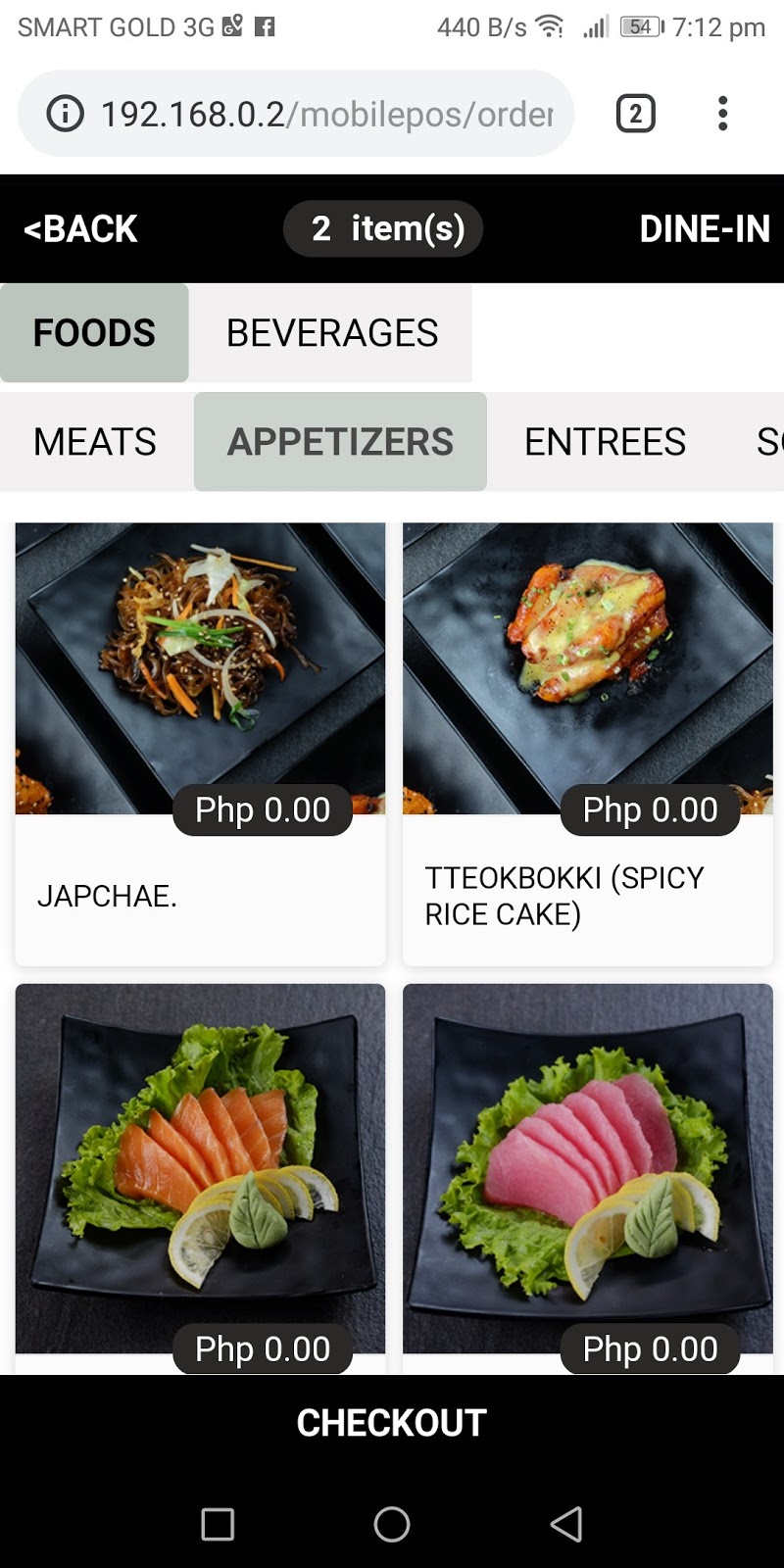This image is a screenshot of a mobile website, viewed on a smartphone. The top header is white, displaying "Smart Gold 3G" on the left and the time "7:12 p.m." on the right, along with a battery icon indicating a 54% charge. Just below the header, the web address is partially visible, showing "192.168.0.2/mobilePOS/order."

A black border separates the header from the main content, which features a white background. The menu is organized in two horizontal rows, listing categories such as Foods, Beverages, Meats, Appetizers, and Entrees in a gray font. The menu buttons are shaded in varying tones of gray.

Below the menu, there are images of four different food items, each presented on a dark bluish-gray square plate. The upper left-hand image is labeled "JAPCHAE," featuring a dish that appears to include noodles, meat, and vegetables. To the right, "Spicy Rice Cake" is shown, looking fried with red coloring. The lower left image seems to depict sushi, with pieces of a more orange hue, and the lower right image also appears to be sushi, but in a pink color.